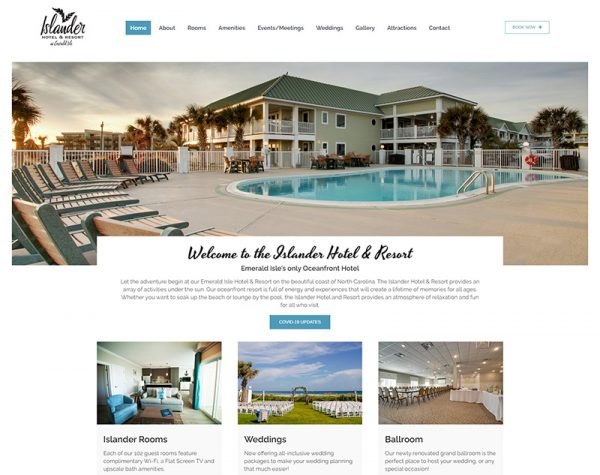The webpage screenshot features a horizontally rectangular frame with a predominantly white background. In the top left corner, the words "Islander, Hotel, and Resort" are prominently displayed. Spanning horizontally across the top, visitors can navigate through various options, including Home, About, Rooms, Amenities, Events, Weddings, Gallery, Attractions, and Contact.

Directly below the navigation bar, a large, horizontally rectangular image showcases the hotel's exterior, complete with a view of the inviting pool area. Centered beneath this main image, a smaller horizontal rectangle warmly welcomes visitors with the text: "Welcome to the Islander Hotel and Resort, Emerald Isle’s only oceanfront hotel." 

Although the subsequent text is difficult to decipher, it provides important details about the hotel. Below this verbiage, a blue button is centered, labeled "COVID-19 Updates," offering crucial information on the current health protocols.

Further down the page, three side-by-side images are displayed. The first depicts the cozy interior of a hotel room, the second shows an outdoor area with neatly lined seating, and the third captures the elegant ballroom. Each image is clearly labeled below, respectively, as Islander Rooms, Weddings, and Ballroom.